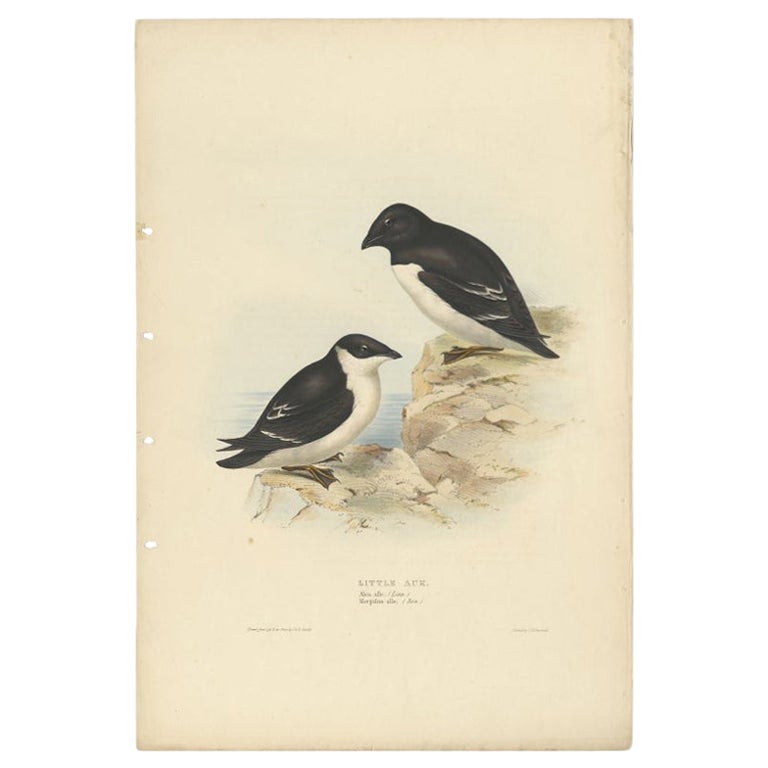An illustration depicts two auk birds poised on a rocky cliff against a serene, light blue sea background. The auk on the left stands on a lower ledge, while the one on the right occupies a higher position. Both birds exhibit a striking black and white plumage, with black tops and white undersides, and they possess webbed feet. The setting features beige and brown rocks signifying a natural habitat. At the bottom of the illustration, there is some barely legible gray text, beleaguered by an ornate cursive font that includes the words "little oak.” The illustration is rendered on a piece of paper punctured by four holes on the left side, enhancing the rustic and vintage aesthetic of the presentation. Overall, the scene evokes a tranquil seaside environment where these short, stocky birds are naturally at home.